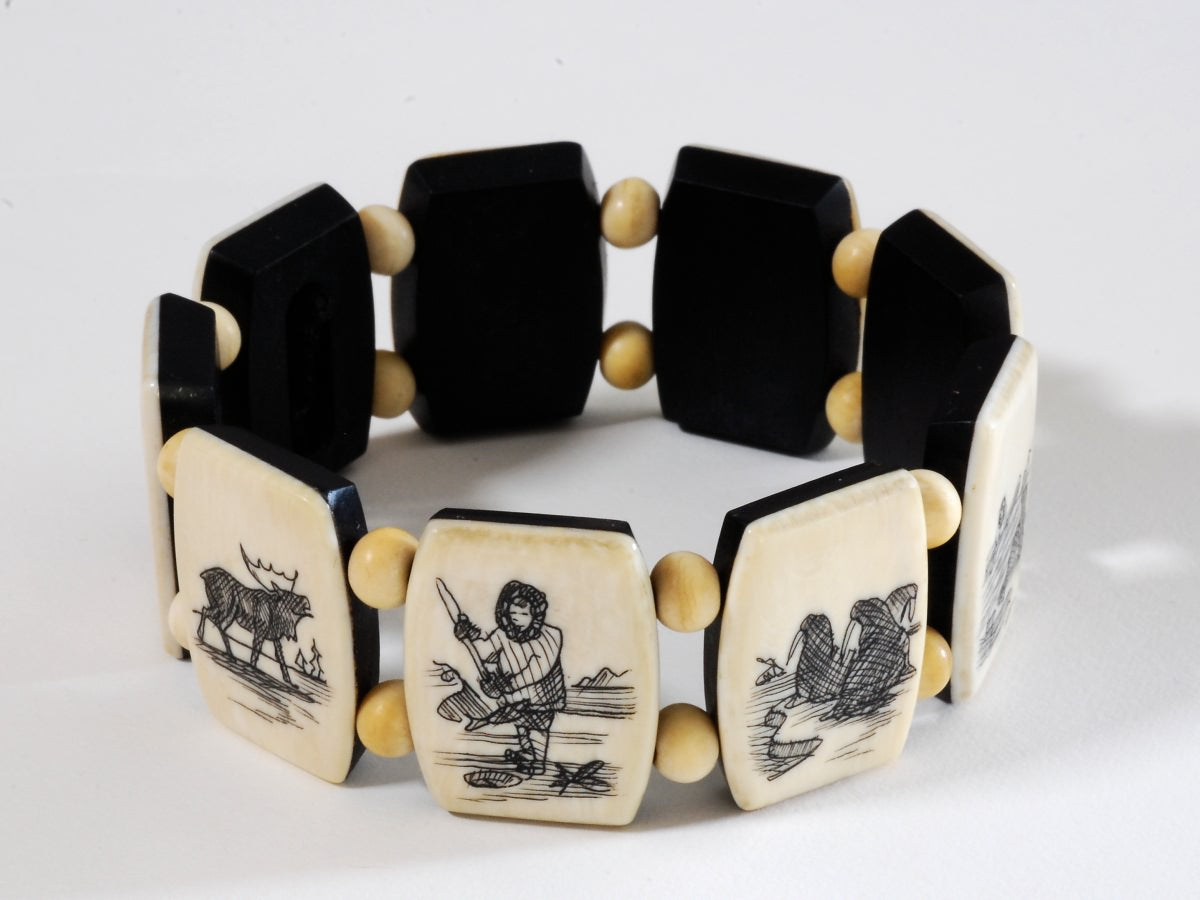This detailed photograph features an intricately handcrafted bracelet, composed of nine lozenge-shaped plates that are four-sided with shorter flat sides on the top and bottom and longer shallow curved sides on the left and right. Each plate appears to be crafted from scrimshawed ivory, with some sections showing a brownish patina indicative of age. 

The foremost plate depicts a finely detailed black line drawing of an Inuk person holding an ice fishing spear in front of a hole, with a horizon line and rocks sketched in the background. The plate to the left showcases an animal resembling an ugulet with prominent antlers, while the plate to the right features two identifiable walruses, distinguishable by their tusks, resting on what appears to be an icy shoreline.

The bracelet is linked together with pairs of yellowish ivory or pearl beads between each plate, contrasting with the black backing of the plates. The entire piece is positioned centrally within a gray background, emphasizing the artisan craftsmanship and cultural symbolism of the images on each plate. The jewelry showcases a palette of ivory white, beige-tan, and black, highlighting the natural materials used in its creation.